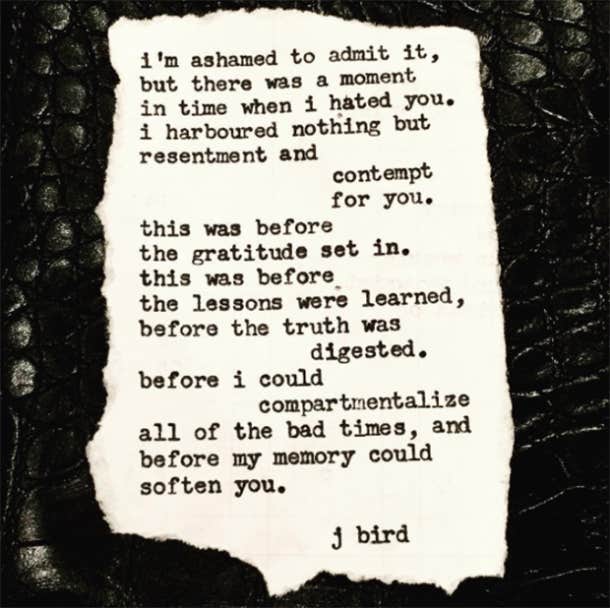In this digitally generated or potentially photographed image, a poignant block of text resembling a typewritten letter or poem is prominently displayed. The text reads: "I'm ashamed to admit it, but there was a moment in time when I hated you. I harbored nothing but resentment and contempt for you. This was before the gratitude set in. This was before the lessons were learned, before the truth was digested, before I could compartmentalize all of the bad times, and before my memory could soften you, J-Bird."

The text is centered vertically within the image, written in black on a white or off-white torn piece of paper. The background appears to be a textured, black leather-like material, possibly resembling alligator skin. The overall color palette consists of black, white, gray, and hints of off-white, creating a stark, monochromatic contrast. This visual composition, with its old-fashioned typewriter style, evokes a sense of nostalgia and emotional rawness. The image's design suggests that it may be intended for digital sharing, such as in an email or on social media.